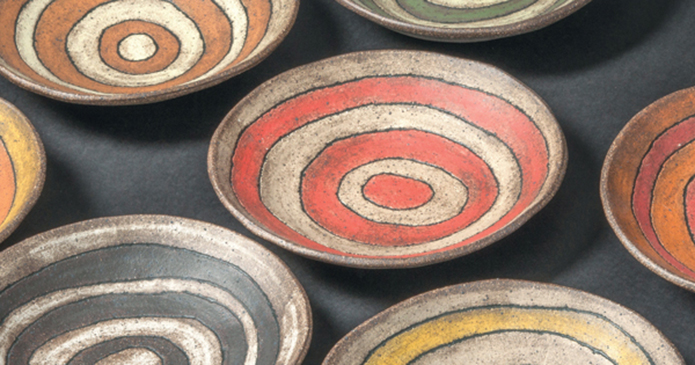The horizontally aligned rectangular image captures a close-up of several vintage, painted bowls or plates artfully arranged on a dark gray surface, likely a table or workshop space. Each of the bowls features a distinctive circular, bullseye pattern that spirals inward from the outer edge, showcasing a variety of vibrant colors including shades of gray, red, orange, yellow, green, black, and white. Only one dish, located centrally, is fully visible; it is gray speckled with brown and exhibits concentric circles in orange. The plates on the periphery are partially visible, with notable examples including: a plate in the upper left with orange and white stripes, one in the lower left bearing gray stripes, another in the lower right adorned with yellow hues, and a partially seen plate on the right featuring a beige and orange color scheme. The bowls' various color combinations and patterns highlight an artistic and vintage aesthetic, all set against a very dark gray backdrop under bright, clear lighting which enhances their intricate details and vibrant colors.